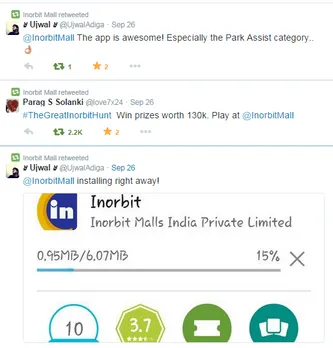The image frame is slightly vertically rectangular in shape. It features multiple small screenshots of retweets. At the top, the text "inorbit mall" is visible, indicating the original source of the retweets. 

In the first retweet, the user "UJWAL" is mentioned, along with their profile icon. This particular retweet praises an app, specifically highlighting the "park assist" category as being "awesome."

The second retweet by "inorbit mall" promotes a contest with prizes worth $130,000 and invites users to "Play at inorbit mall."

In the third retweet, "UJWAL" appears once again, sharing their enthusiasm about the "inorbit mall" app installation. A screenshot accompanying this retweet shows the download in progress, detailing "Inorbit Malls India Private Limited" with a progress bar indicating 0.97 megabytes out of 6.07 megabytes downloaded, equating to 15% installation completed.